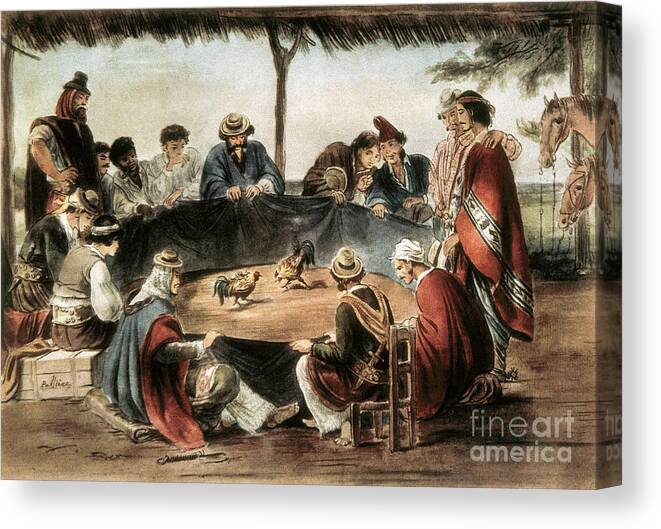The image depicts a detailed, primitive-style illustration set in what appears to be Mexico or the southwestern United States. The scene is of an outdoor cockfight viewed from slightly elevated, straight-on perspective. Underneath a thatched grass roof, men and women dressed in various robes, predominantly in shades of red and blue, gather in a circle around a central ring. They hold up a fabric circle, focusing their attention on two roosters engaged in a duel. In the background, two horses are either tethered or watching the spectacle. The environment suggests an open-walled, porch-like structure with a dirt floor. The artwork has a dated feel, reminiscent of the 16th or 17th centuries, rendered in earthy tones including browns, sepias, grays, beige, blue, and red. In the bottom right corner, the text "Fine Art America" is visible, indicating the image wraps around a canvas.